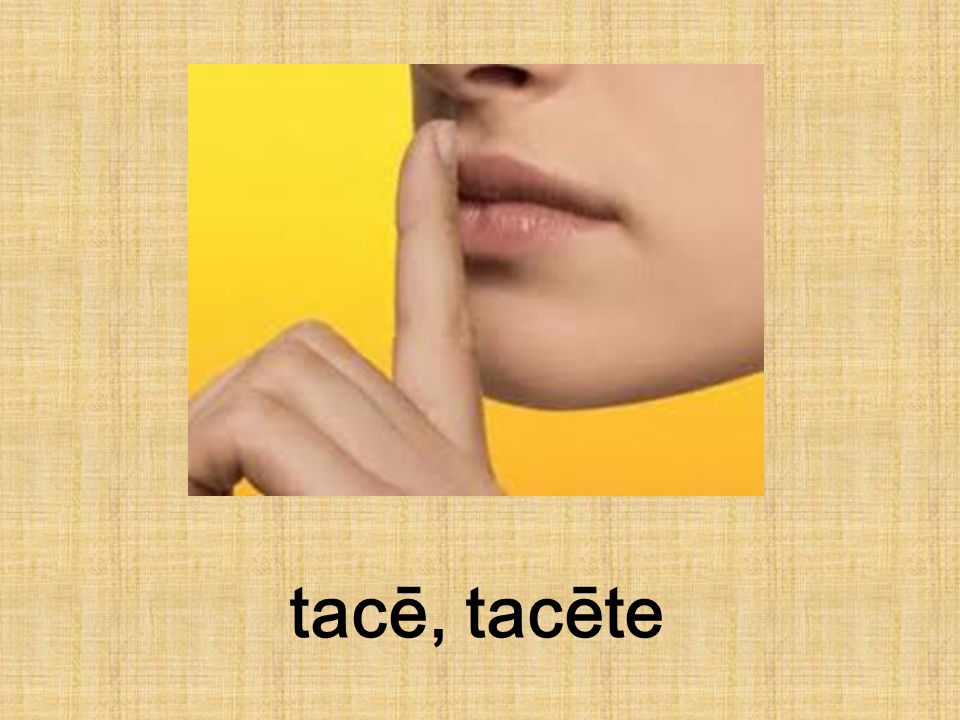The image is an educational slide featuring a close-up photograph of the bottom part of a person's face, specifically the area from the nose to the chin, with their index finger placed vertically across their lips in a universal "shush" gesture. The other three fingers are folded down. The inset photo has a light yellowish-orange background, distinct from the overall slide, which features a beige, grass-cloth-like pattern with a checkered texture. Below the photograph, in black lowercase text, are the words "tace, tacete," likely indicating instructions to be quiet in a foreign language. The slide's overall border has an orange hue, tying in with the color scheme of the inset photograph's background.